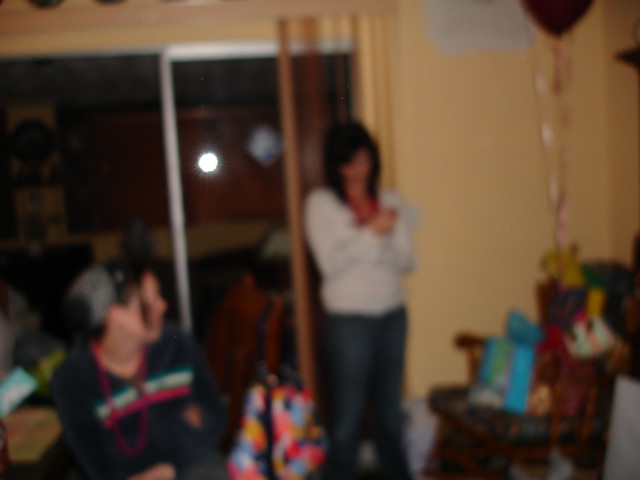The photograph, framed slightly wider than tall, captures a moment in what appears to be an intimate, yet blurry interior setting, possibly a birthday party or a celebration. On the right side of the image, a portion of a yellowish-tan wall is visible, contrasting with a large sliding glass door with a silver frame on the left side. The glass door hints at an external environment that remains out of focus. 

In the upper right corner, the base of a balloon with a ribbon dangling suggests a festive atmosphere. Central to the composition, a figure stands facing the camera, though their gaze is directed downward. This individual is characterized by long black hair, a white shirt, and dark blue pants, potentially jeans, though the blurriness obscures finer details. 

To the right, another person is partially captured from the waist up, seemingly seated. This individual wears a bandana over their head, with a loose strand of hair hanging across their cheek as they look off to the right. Their attire consists of a dark blue or black long-sleeve shirt adorned with two horizontal stripes across the chest—light blue on top and red below. 

The haziness of the image imparts a sense of motion or perhaps a nostalgic, dreamlike quality, emblematic of cherished moments fleetingly preserved.